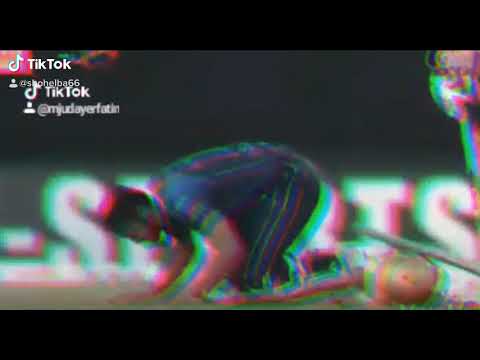This is a screenshot from a TikTok video captured during a soccer game. The image features a man in a dark blue jersey with green, blue, and red stripes on the sleeves, and matching soccer shorts adorned with red, blue, and yellow stripes along the sides. He is on his hands and knees on what appears to be a soccer pitch, possibly with a ball nearby. In the top left corner of the screenshot, the TikTok logo and the word "TikTok" are visible along with the handle "@MJUDAYERFATHIN" and a profile image, though another handle "@SHOHELB-A-66" is also faintly visible. The background includes letters that seem to spell out "sports" alongside a fence marking the side of the field. The overall image is somewhat blurry, highlighting the chaotic yet dynamic moment captured in the sports setting.